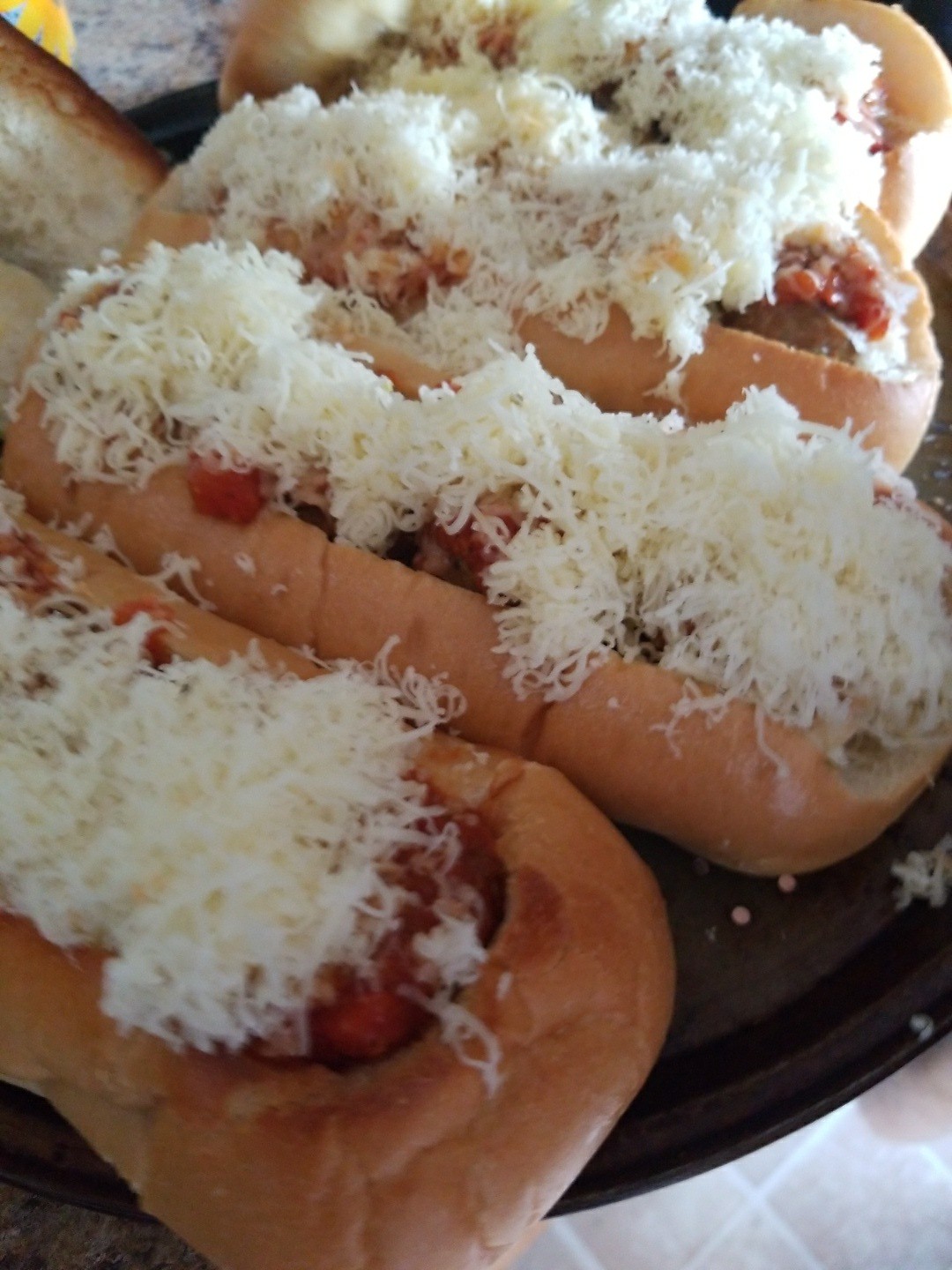This is a close-up, slightly blurry color photograph of a plate holding four sandwiches. The sandwiches are laid out on a black plate, which appears to rest on a countertop with beige tile flooring visible in the bottom right corner. Each sandwich comprises a hoagie-style bun that's hollowed out to form a boat-like shape. The buns aren't toasted and hold a filling that seems to be a chunky marinara sauce with possible meatballs and minced tomatoes or peppers. The filling is generously topped with mounds of finely shredded white cheese, which is not melted. To the top left corner of the image, there is an additional piece of toasted bread. The overall appearance is of substantial, cheese-covered sandwiches, possibly meatball subs, rather than hot dogs.